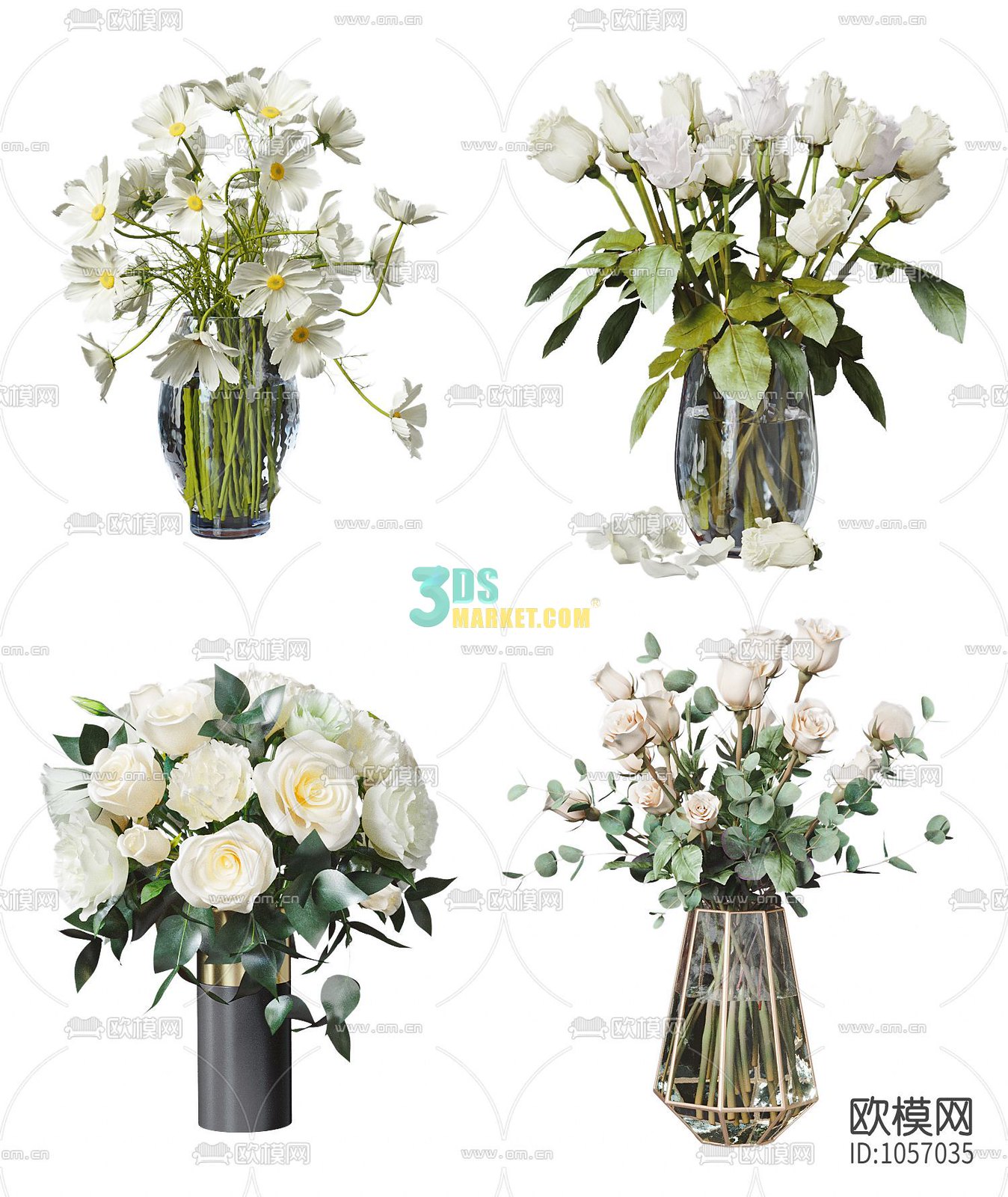The image is a color photograph designed to resemble an advertisement for a florist, featuring four distinct flower arrangements, each in a unique vase. In the top left, white daisies with yellow centers are arranged in a clear vase, displaying green stems. The top right holds tightly closed white roses, also with noticeable green foliage, in another clear vase. The bottom left shows fully bloomed white roses in an elegant black vase adorned with a gold stripe. The bottom right features a geometric, clear vase with pale pink flowers and a hint of eucalyptus leaves, providing a delicate, sophisticated touch. A watermark with the text "3dsmarket.com" is visible, along with some writing in a different language, suggesting the image may have been sourced from a website.